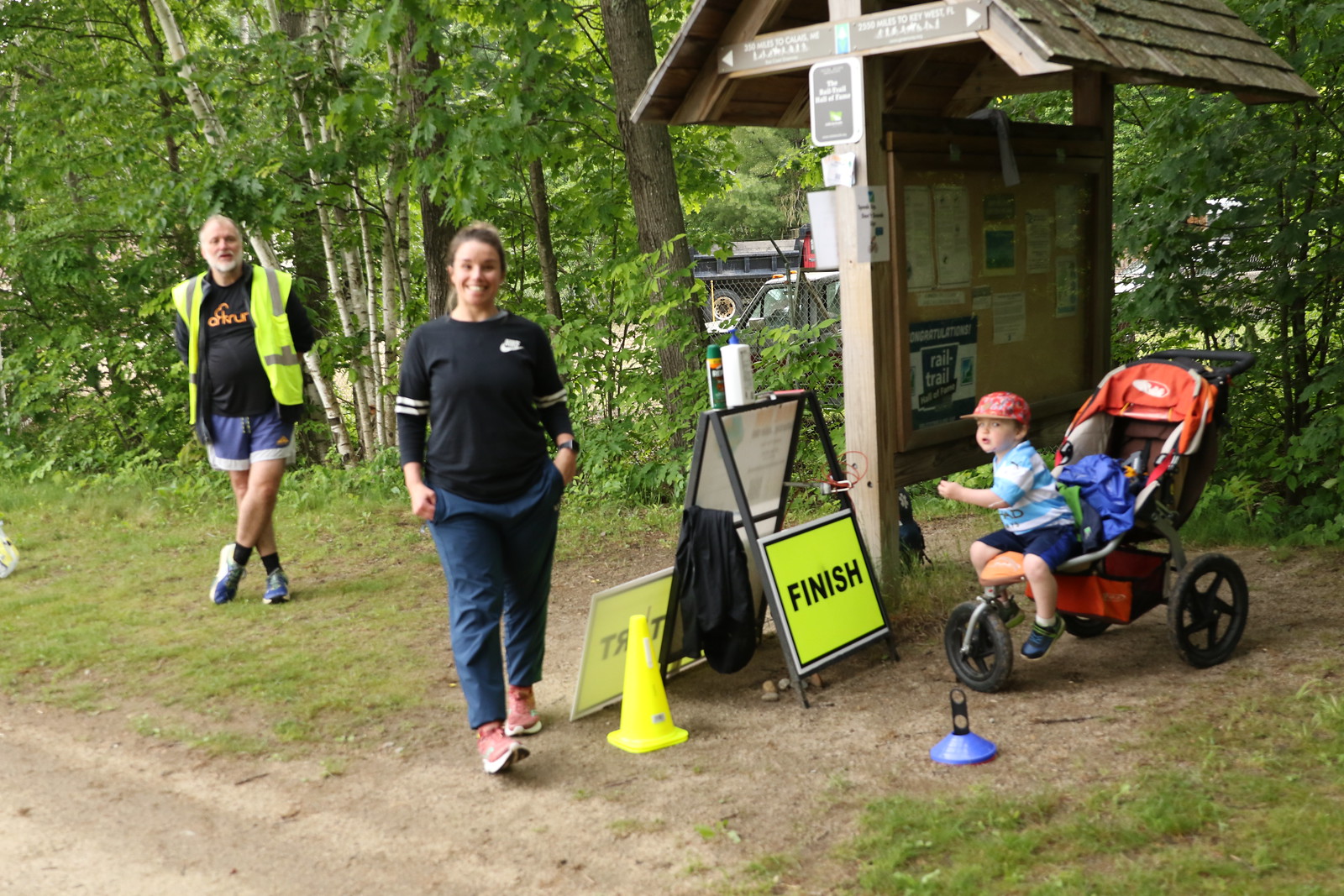In a lush park setting with abundant greenery and trees, a cheerful lady stands prominently in the center, smiling brightly. She is dressed in a black long-sleeved shirt with white detailing on the arms, blue pants, and pink shoes, and she has her hands tucked into her pockets. To her. left is an older gentleman with white hair and a beard, clad in a black shirt with orange writing, covered by a bright yellow reflective vest. He is also wearing navy shorts, black socks, and navy running shoes, standing with his feet crossed and hands behind his back. To the right of the lady is a vibrant yellow sign marked "finish," set up on a tripod, accompanied by a small yellow safety cone. Beyond the "finish" sign stands a wooden shelter with a distinctively shaped roof; beneath it lies a bulletin board with glass covering, showcasing various posters. Just to the right of the shelter is a bright orange and red stroller occupied by a young boy about two years old. He wears a red hat, a light blue and white striped shirt, blue shorts, and dark-colored shoes, and sits happily in his stroller. The background reveals a mixture of trees and bushes, completing this scenic outdoor gathering.